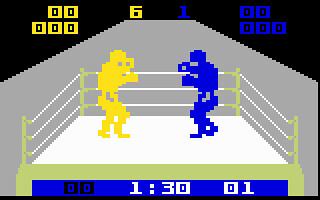This image is a screenshot from a pixelated, old-school video game depicting a boxing match between two rough, humanoid shapes resembling robots or Lego characters. The left figure is yellow, and the right figure is blue, both inside a three-sided boxing ring with white ropes on three sides, leaving the front open to our view. The ring has a white and mint green color scheme, featuring a white floor and green frame. The top of the image includes a black border, within which sits the scoring area: six yellow blocks on the left, indicating the score for the yellow character, and one blue block on the right for the blue character. This also seems to indicate remaining lives, five for each combatant. A blue banner at the bottom displays a timer with "1:30" in white, possibly indicating the time elapsed or remaining in the bout, flanked by indicators "00" and "01" as well. The background contrasts with a nicely lit ring against a dark backdrop, emphasizing the arena and figures within it.